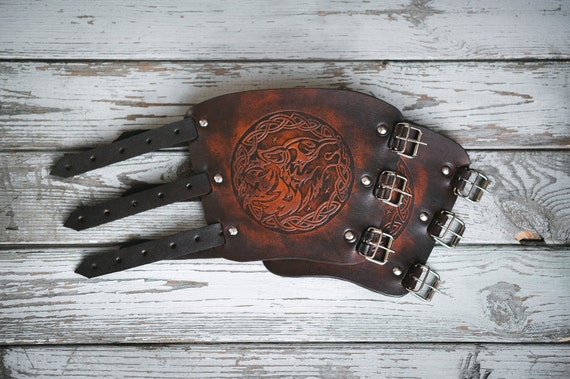The image features two intricately designed leather wristbands resting on a gray, wooden surface. The wristbands are primarily black with striking orange accents, creating a visually appealing contrast. Each wristband has a distinctive circular emblem embossed into the leather, adding an element of uniqueness and style. To the left side of the image, three black straps with metal snaps are visible, designed for securing the wristbands comfortably around the wrist. The layered positioning of the wristbands, with one placed atop the other, along with the rustic backdrop, enhances the artisanal and rugged aesthetic of the scene.